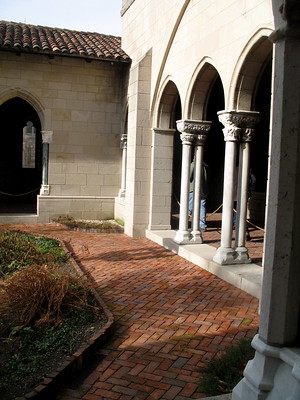The image features an outdoor courtyard dominated by a brick walkway adorned with various shades of red bricks arranged in a distinctive pattern, angling to the right, proceeding straight, and then bending towards the left. On the left side of the walkway lies a garden area consisting of a mix of green and brown plants, situated in a raised planter bordered by bricks. The background showcases a white brick building with a cathedral-style façade. The building features a distinct door embedded within a cathedral-like archway and a brown tiled roof. The right side of the building is taller and displays three evenly spaced arched openings, each flanked by pairs of intricately decorated columns, resembling a classical Roman or Greek architectural style. These columns are designed with spaces between two rods, and the archways extend into a frame that accentuates the church-like pattern of the structure. The predominant colors in the scene are white and orange, which complement the antique, almost reverent ambiance of the courtyard.